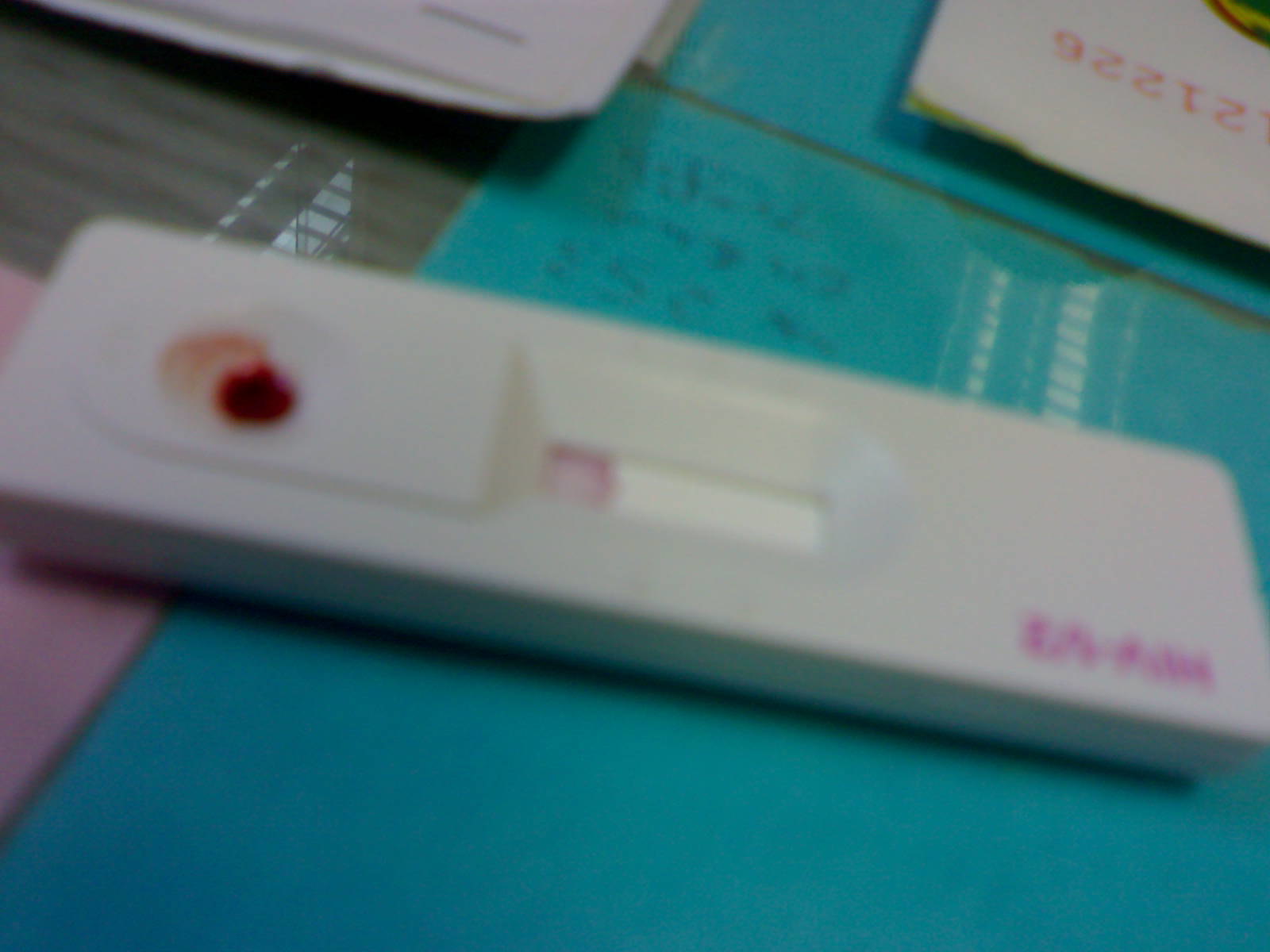The photograph depicts a poorly focused scene centered around a blood test setup. In the foreground, a recent drop of blood is visible on the left side of the white test apparatus, which features small pink letters on the bottom right—too blurry to discern clearly. The test sits atop a blue sheet of paper with illegible writing, flanked by partially visible white papers at the top and a pink paper slightly to the left.

The table beneath the setup is the sharpest element in the image, displaying a reflective surface that captures the ceiling’s metallic struts and detailing. The table, although comprising less than 10% of the frame, becomes the visual focal point due to the camera's misaligned focus. This unintended shift directs the viewer's attention away from the intended subject—the medical test—and towards the sharply rendered table and its reflection.